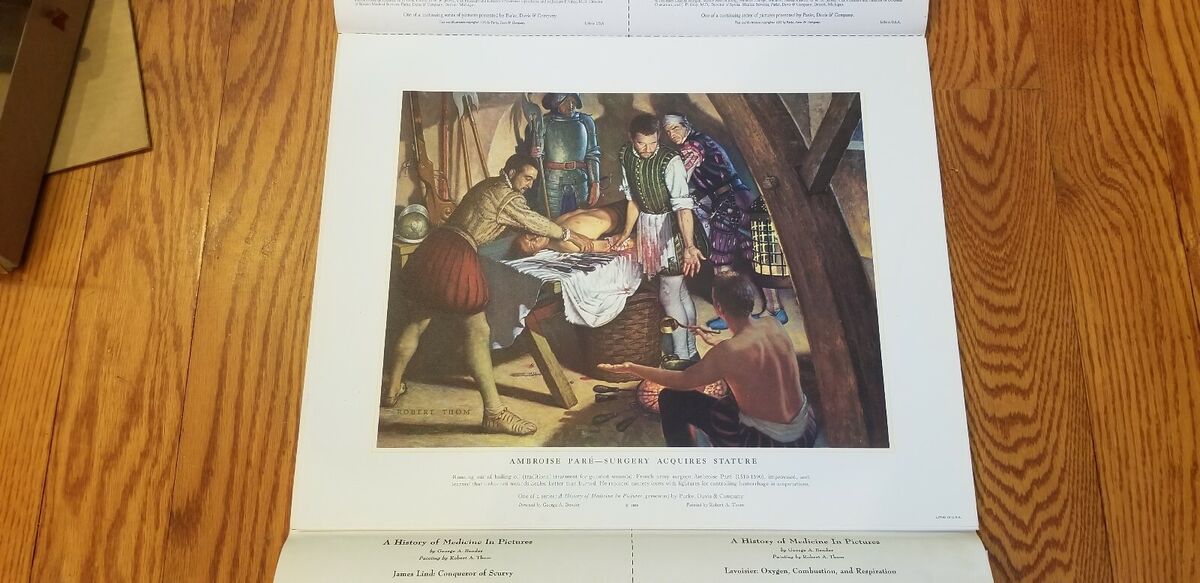This photograph captures a piece of classical artwork printed on a white sheet of paper, which lies on a light brown wooden table with darker brown swirls. Shot from above, the paper features black text underneath the artwork, specifically the caption "Ambrose Paret's Surgery Acquires Structure." The scene depicted in the painting is a dramatic surgical procedure. At the center, a man with his shirt off is restrained on a table draped with a white cloth. To his right, a figure in a beige top and red skirt holds his arm, while opposite him, another man in a green vest with rolled-up sleeves aids in the restraint. A soldier in metal armor stands prominently behind them, wielding a spear. In the foreground, another shirtless man with black pants sits on the floor, watching intently. Two additional men, one armed with a dagger, are seen in the background observing the procedure. The piece of paper is slightly curved upwards at the top and bottom edges.